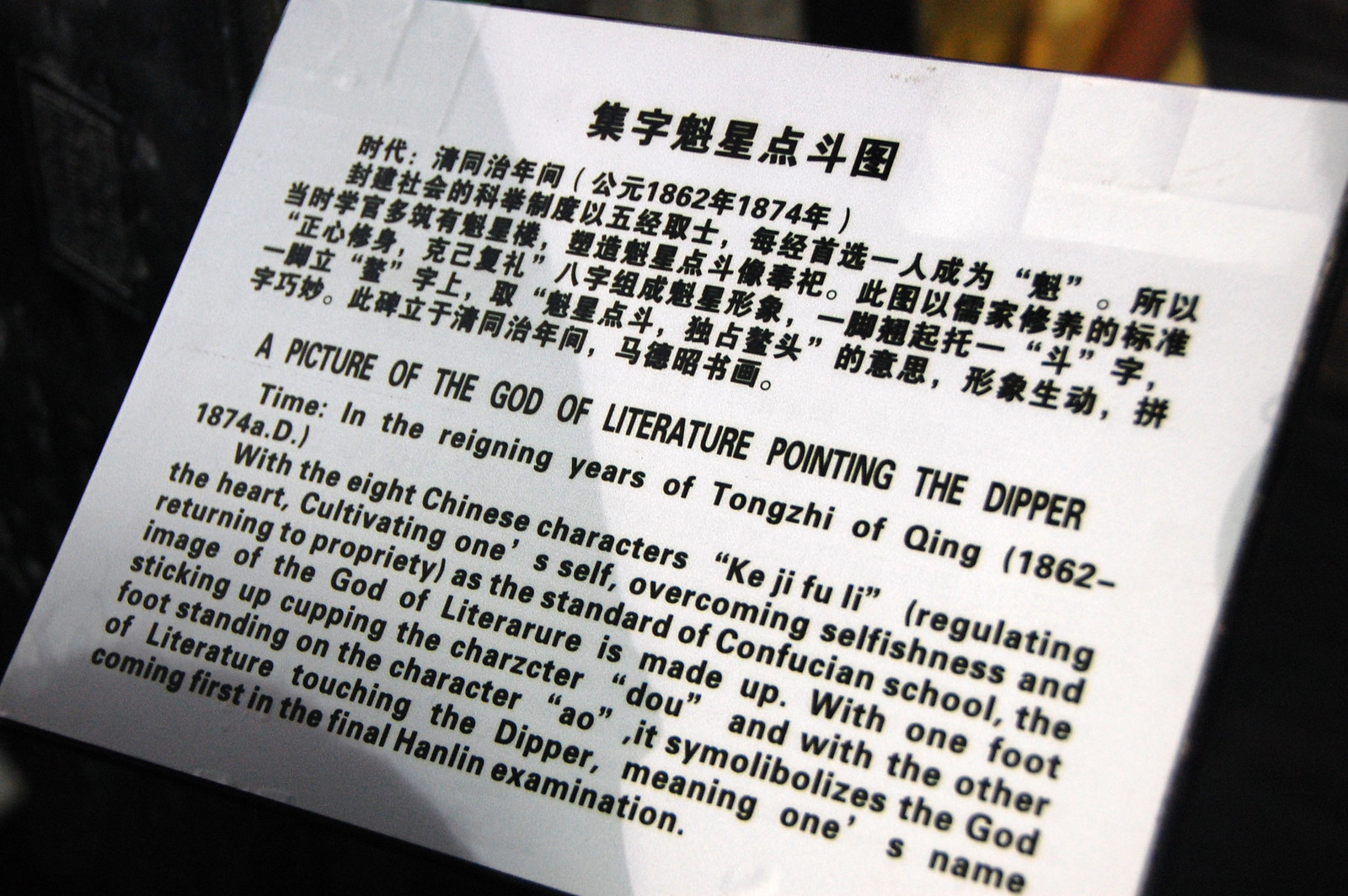The image displays a single object, likely a sign, poster, or card, positioned prominently in the center of the frame. Set against a dark, blurred background, the object features both Chinese characters and English text. The top section contains several lines of thick, black Chinese writing. Beneath this, bold capitalized English text reads: "A picture of the God of Literature pointing to the Dipper. Time in the reigning years of Tongzi of Qing, 1862 to 1874 AD." Following this is a detailed English description: "With the eight Chinese characters regulating the heart, cultivating one's self, overcoming selfishness, and returning to propriety as a standard of Confucian school, the image of the God of Literature is made up with one foot sticking up, cupping the character Du, and with the other foot standing on the character Ao. It symbolizes the God of Literature touching the Dipper, meaning one's name coming first in the final Hanlin examination." The colors visible within the image are predominantly black, white, and brown, suggesting that the photograph was taken indoors in a dimly lit room.